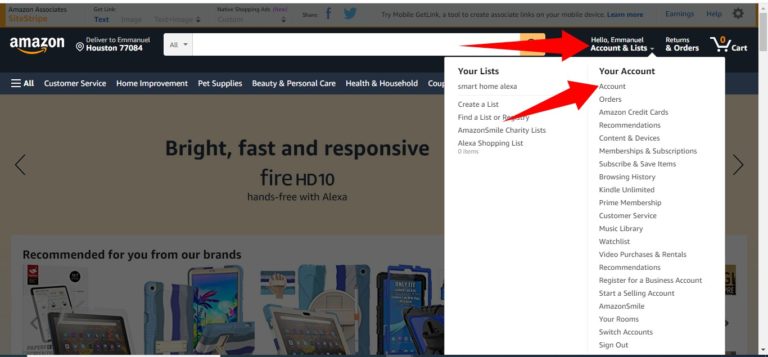This screenshot captures the Amazon.com homepage, presented in a tutorial-like format with a slight gray filter overlay. A prominent white pop-up menu occupies the center of the screen, highlighted by two red arrows for emphasis. The pop-up menu, displayed in black font, outlines various functionalities under two main headings. The first section titled "Your Lists" includes options such as Smart Home, Alexa, Create a List, Find a List or Registry, Amazon Smile Charity Lists, and Alexa Shopping Lists. 

The second red arrow points to the "Your Account" section on the right, detailing a comprehensive list of account-related options. These include Your Account, Orders, Amazon Credit Cards, Recommendations, Content and Devices, Memberships and Subscriptions, Subscribe and Save Items, Browsing History, Kindle Unlimited, Prime Memberships, Customer Service, Music Library, Watch List, Video Purchases and Rentals, Recommendations, Register for a Business Account, Start a Selling Account, Amazon Smile, Your Rooms, Switch Accounts, and Sign Out.

At the top of the pop-up menu, another red arrow directs attention to the "Hello, [User], Accounts and Lists" area, indicating where users can access their account settings and lists. This visual guide aims to assist users in navigating key features of their Amazon accounts efficiently.